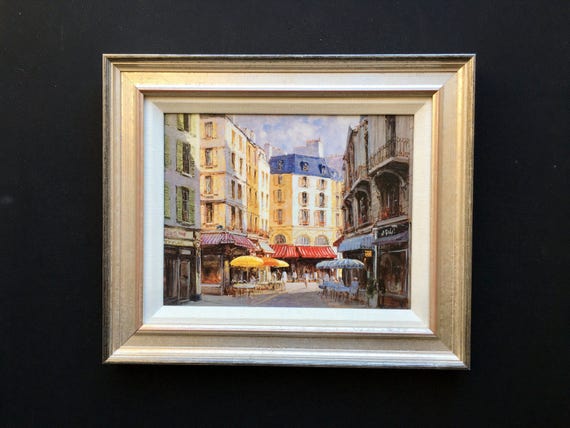This photograph depicts a watercolor painting of a vibrant European street scene, prominently showcasing tall, multi-story buildings (ranging from four to five stories) adorned with numerous windows. The diverse architecture is accented with colorful details: a mostly white building with a blue roof, dark gray structures, and another building with a red roof seen towards the back. Each building is intricately designed, with shopfronts at street level sheltering under various colored parasols—blue on the right side, paired with a matching canvas, and yellow on the left. Red cabana-style awnings further add to the lively ambiance.

The street is bustling with people enjoying their day, adding life to the scene. Above, a patch of blue sky peeks through, dotted with white clouds and casting light down the central alley between buildings. This atmospheric painting is encased in a natural wood frame with a light gold hue, mounted against a stark black wall, drawing attention to its detailed and colorful depiction of urban life.